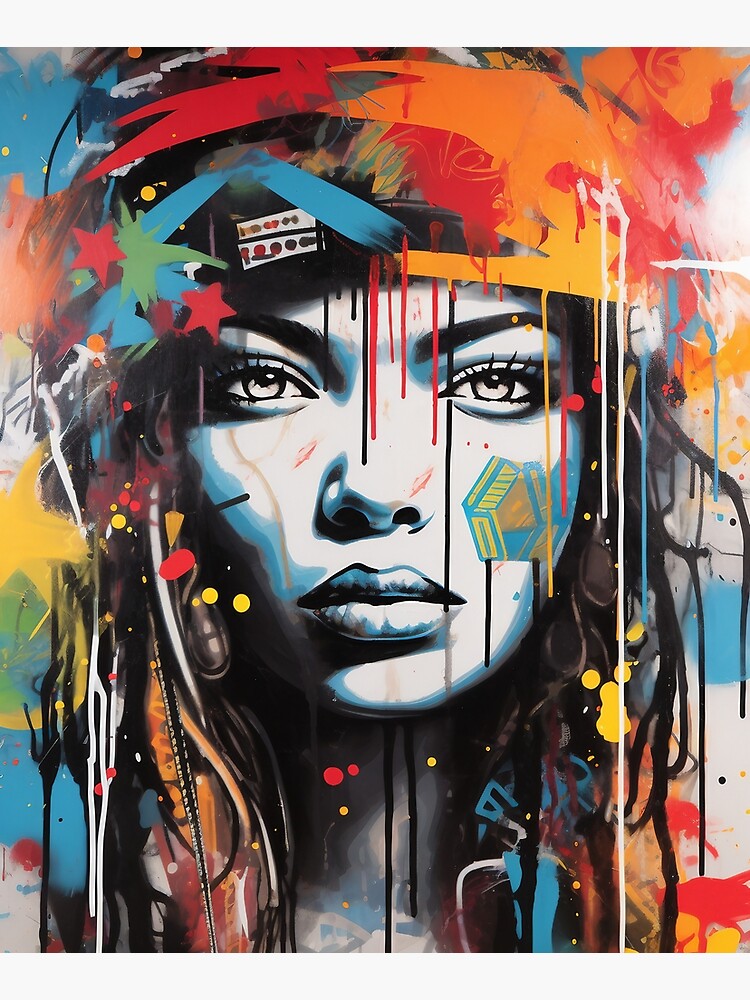The painting portrays a young woman with facial features that suggest she might be a black woman, such as full lips and a distinct facial structure. Her face, rendered in white and various shades of light blue, stands out against her dark hair. The style is reminiscent of a comic book, with a posterized effect that emphasizes color bands over gradients. Intricately entwined in her hair are streaks and dribbles of paint, creating a vivid, almost headdress-like appearance with bright splotches of yellow, red, orange, and blue. Some of these colors also form geometric patterns, possibly resembling a temporary tattoo on her cheek in blue, yellow, and orange. The woman wears a headband beneath these artistic paint effects, contributing to the intricate design. With her serious, almost fierce expression, she gazes into the distance, giving off a modern, abstract, and dynamic aura. The artwork combines elements of splattered and dripped paint, along with intentional lines, stars, and perhaps even feathers, making it a striking piece suitable for display.